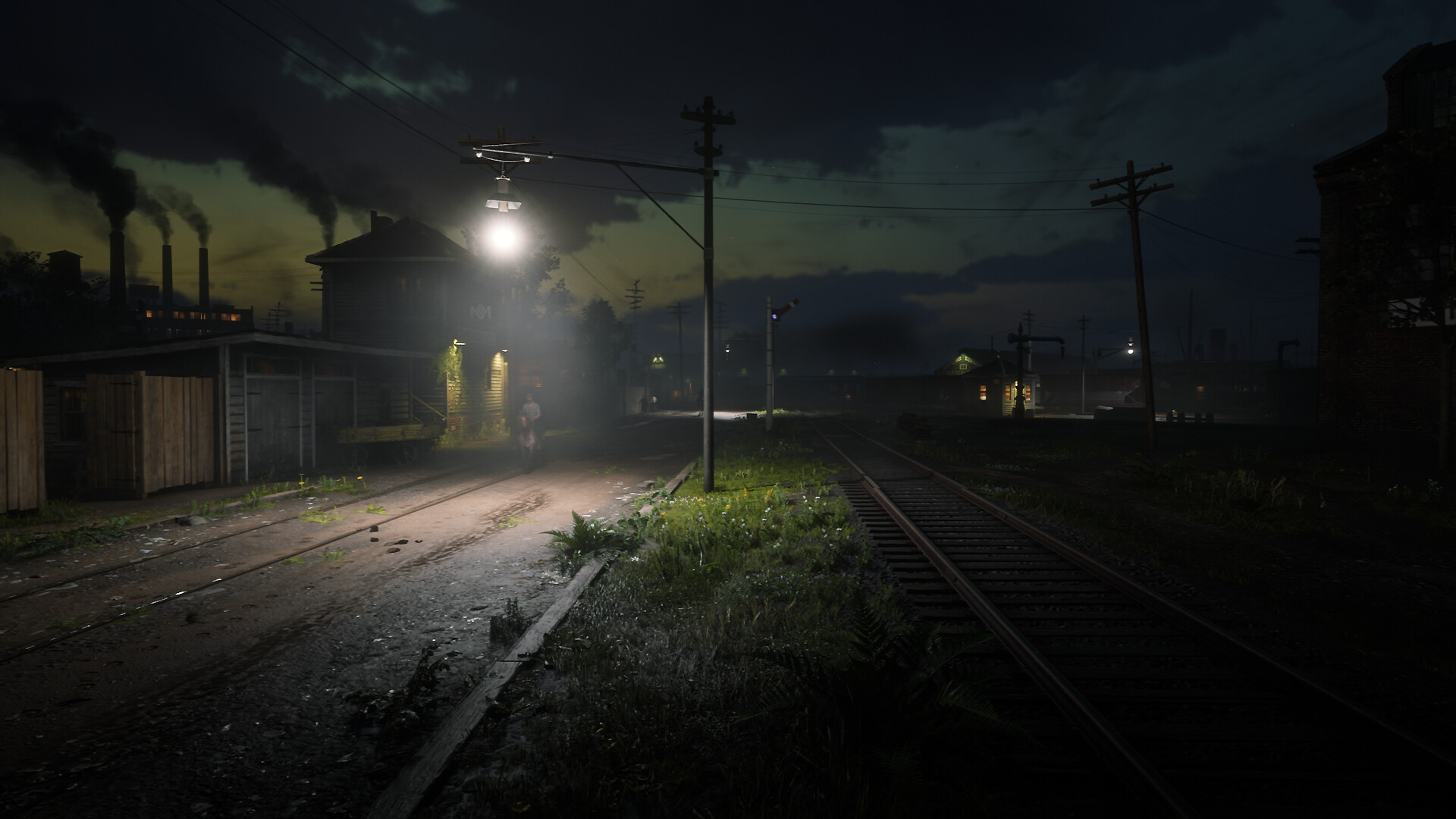This nighttime photograph captures a rail yard scene illuminated by a bright white street lamp perched on a black pole. On the right side, dark brown and black train tracks run parallel to a light brown and dark gray dirt road. The road is bordered by patches of dark green grass. In the foreground, an individual in a short-sleeved gray shirt is riding a motorbike. To the left of the person, an old gray building with illuminated windows and a gray garage-like structure stands near a dark brown fence. In the distance, factories with billowing smoke and glowing windows loom against the partially cloudy sky. The sky, transitioning from a muted orangey-brown near the horizon to a smoky blue further up, indicates the remnants of daylight after sunset, while the silhouettes of clouds add a moody atmosphere to the scene. A row of lights on buildings lines the far right side, complementing the dark green grass below.